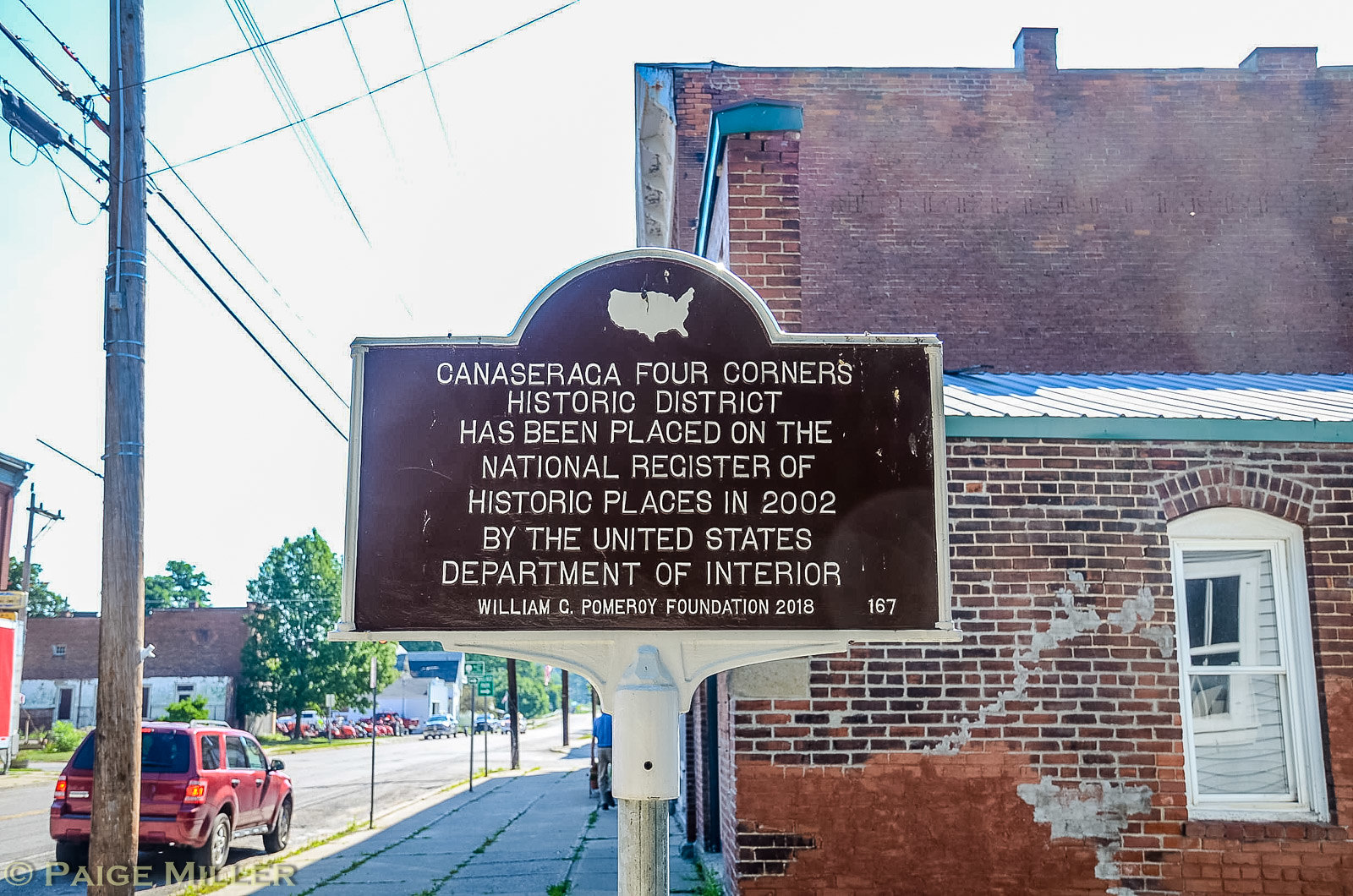The daytime photograph centers on a historical sign situated on a sidewalk in an American town, evidenced by the curved section of the sign that features a silver map of the United States. The sign, which is brown with a silver border, reads in silver text: "Canasaraga Four Corners Historic District has been placed on the National Register of Historic Places in 2002 by the United States Department of the Interior. William C. Pomeroy Foundation 2018." This sign marks the historical significance of the district in view. In the background, there's a brick building with visible repairs where individual bricks have been covered by repair materials. A red SUV is parked outside the building, which has a window with white framing and glass. The overall scene suggests the historic district might be somewhat run-down.